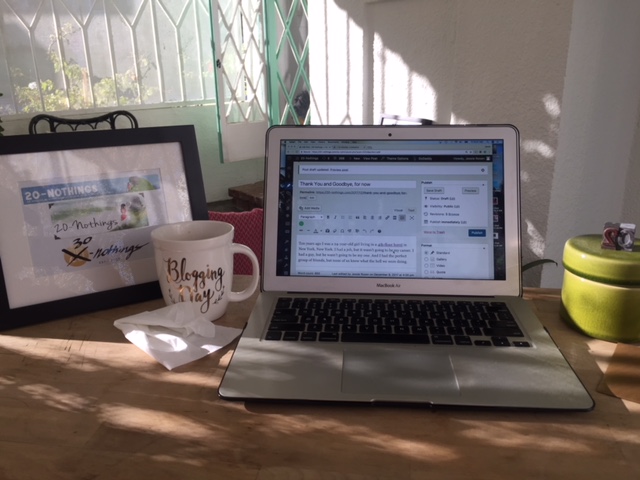In the image, we see a grey laptop with a black keyboard placed on a brown desk. The laptop screen displays a webpage, though the text is too small to be readable, giving it the appearance of a grey and white background. Adjacent to the laptop, on the right, sits a lime green pot. Behind the laptop, there is a white wall partition. On the left side of the image, there's a window featuring a white door with intricate white bars arranged vertically and some in a Y formation, along with X patterns on the door. This wall has a slight green coloring at the bottom. To the far left, a black-framed picture with a white background is displayed, showing a blue line across the middle and a lighter blue square beneath it; the wording on the picture seems to say "20-nothing." 

Additionally, a white porcelain mug with gold or bronze lettering reading "Blogging Day" sits beside the laptop. In front of the mug, partially underneath it, there's a white piece of paper. Finally, a red object, possibly a pop, is visible behind the mug, positioned against the wall.